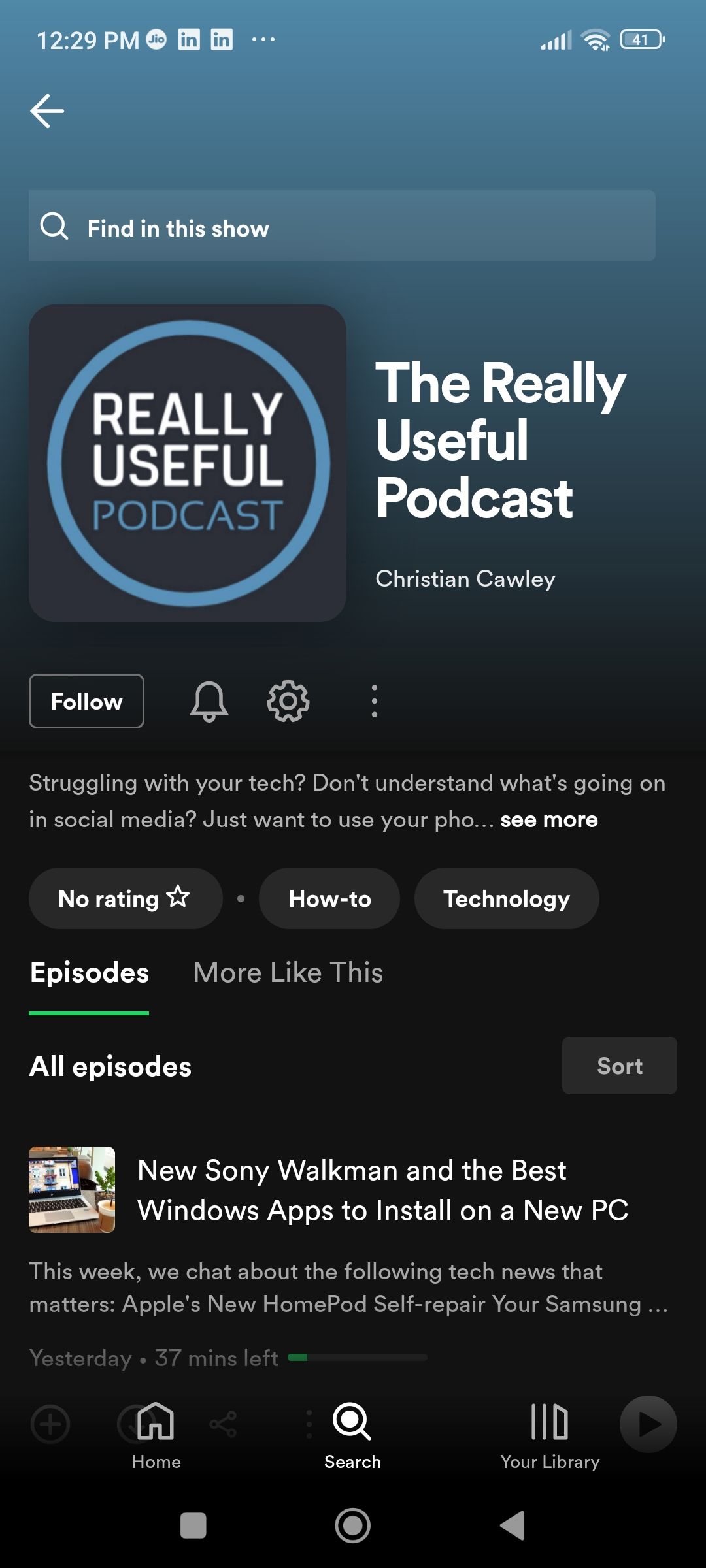Screenshot of a mobile device screen displaying a podcast interface.

### Detailed Description:

- **Background**: The screen features a gradient background transitioning from medium blue at the top to black at the bottom.
- **Time & Status Indicators**: 
   - At the very top, the status bar shows the current time as "12:29 p.m."
   - Following the time, there are three small icons and three dots.
   - On the right side of the status bar, it displays three bars of signal strength, a Wi-Fi symbol, and a battery icon.

- **Navigation & Search**:
   - Below the status bar, there's a left-pointing arrow, indicating a back function.
   - Next to the arrow is a search bar, which is a slightly lighter shade of gray and includes a magnifying glass icon on the left side.

- **Podcast Information**:
   - Centered on the screen is a square image with the text "Really Useful" in white letters, placed on a blue background with a blue circle.
   - To the right of this image, the podcast title "The Really Useful Podcast" is displayed prominently, with the name "Christian Cawley" written in smaller letters beneath it.
   - Below the podcast title, there are three buttons: "Follow," "Notification," and "Settings."
   - Three vertical bars are present below these buttons.

- **Content & Navigation Tabs**:
   - Below the buttons, a paragraph provides information about the podcast.
   - Following the paragraph, three circular tabs or icons are visible.
   - Below these, a navigational section reads “Episodes," "More Like This," with a green underline indicating "Episodes" is the selected tab.

- **Additional Content**:
   - At the very bottom of the screenshot, there's another piece of content or article visible, though partially cut off.

This detailed description provides a comprehensive overview of the elements and layout of the screenshot, providing clear insight into the interface and features displayed.